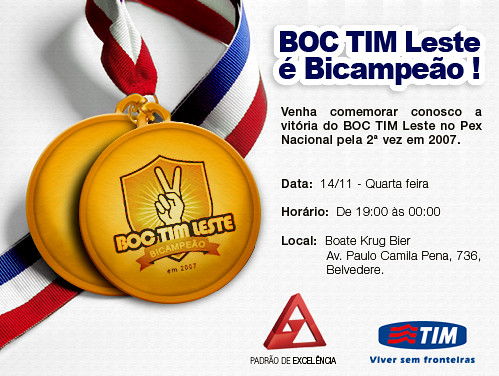The image is a detailed graphical design advertising a sporting event. Against a grey background, it features a meticulously rendered illustration of two gold medals attached to a vertically striped ribbon in blue, white, and red. The ribbon, with a canvas texture and shadow effect, enters from the bottom left corner, loops near the top left, and descends toward the center. The medals, coin-shaped and golden, have a lighter gold background. Prominently, the foreground medal displays a darker gold shield with a hand making a peace sign and the lettering "Bach Tim Lest" underneath.

To the right of the medals, the text, written entirely in Spanish, begins with a dark blue headline with a white drop shadow reading "Bach Tim Lest E.B. Campeau." Following the headline is a paragraph of black text detailing the event, including the date (14/11 quarta fara) and time (Horario: D. 1900 S. 0000). The location is listed as "Local: Boat Krug Bier, Av. Paolo Camilla Pena, 736, Belvedere." The bottom right corner showcases two sponsor logos: a red triangular one labeled "Pedreo D. XL Encia" and a blue oval one marked "Tim" featuring three red wavy lines and the motto "Viver Sem Fronteras" in blue. The harmonious blend of photographic illustration and graphic design gives the image a vibrant and engaging appearance.